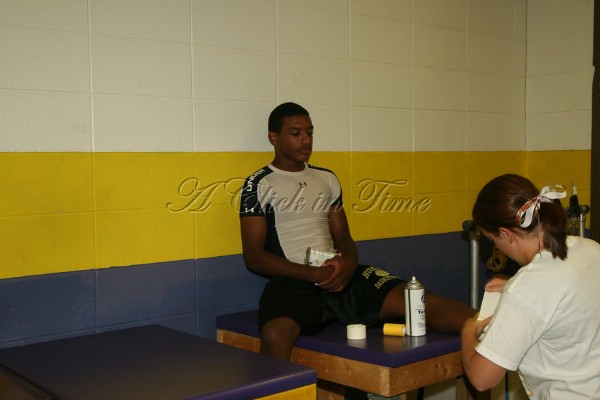In a brightly lit, multi-colored room within what appears to be a backstage area of a sports facility, a young African-American male athlete, likely in his late teens or early twenties, sits on a padded wooden training table. He is wearing a white and black spandex shirt and black shorts which bear a logo on the left side. His leg is extended and propped up, indicating he is receiving medical attention. Next to him is a woman with her back to the camera, dressed in a white shirt and wearing a gold ribbon in her hair. She appears to be applying a bandage to his knee or shin, with an open antiseptic spray and a roll of yellow medical tape visible nearby. The background features a block wall painted in horizontal stripes of white, yellow, and blue, enhancing the clinical atmosphere of the scene. An overlay on the image reads, "A Click in Time."